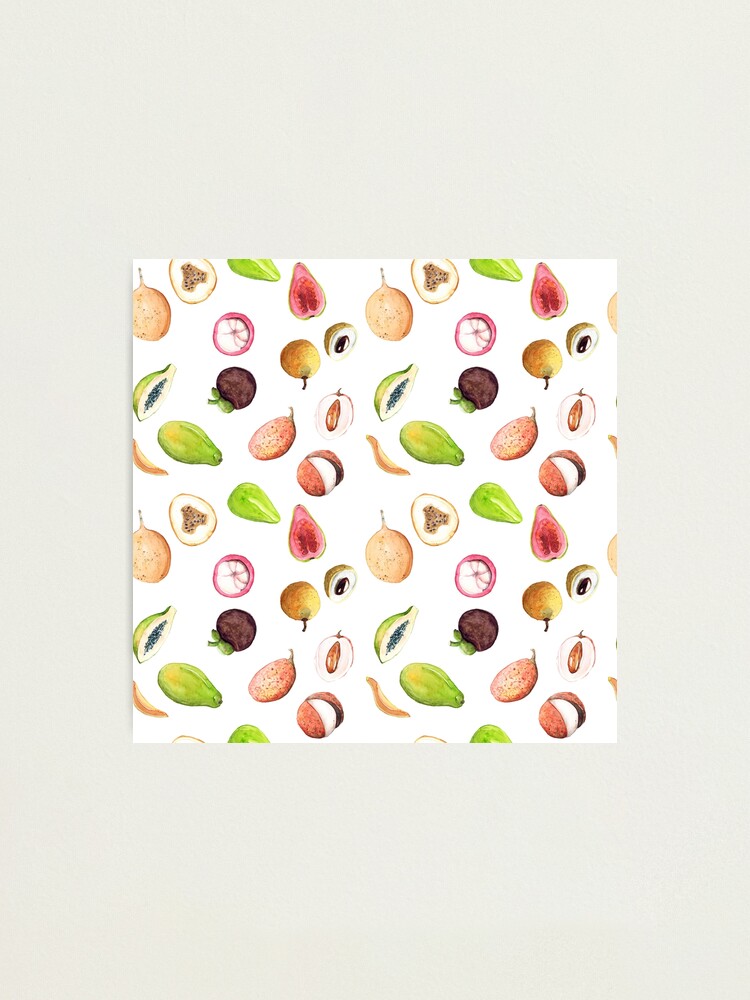This rectangular image, set on a beige background, features a taller-than-wide composition with a central, square white canvas. Adorning this canvas is a decorative pattern of vividly colored fruits painted in a detailed, oil painting style. Principal among these are greenish, pear-shaped and rounded oval fruits, resembling pears and other similar fruits, some of which are depicted both whole and cut open to reveal seedy interiors. A purple, round fruit with green stems suggests the shape of a plum. Peculiar, onion-like fruits stand out, displaying pink rings and lighter inner flesh. The canvas also features coconut-like fruits, brown on the outside and white inside, and mysterious heart-shaped fruits with dark seeds. This detailed and repeated fruit pattern is intricately arranged against the white canvas, juxtaposed against the gray hue of the main image background.